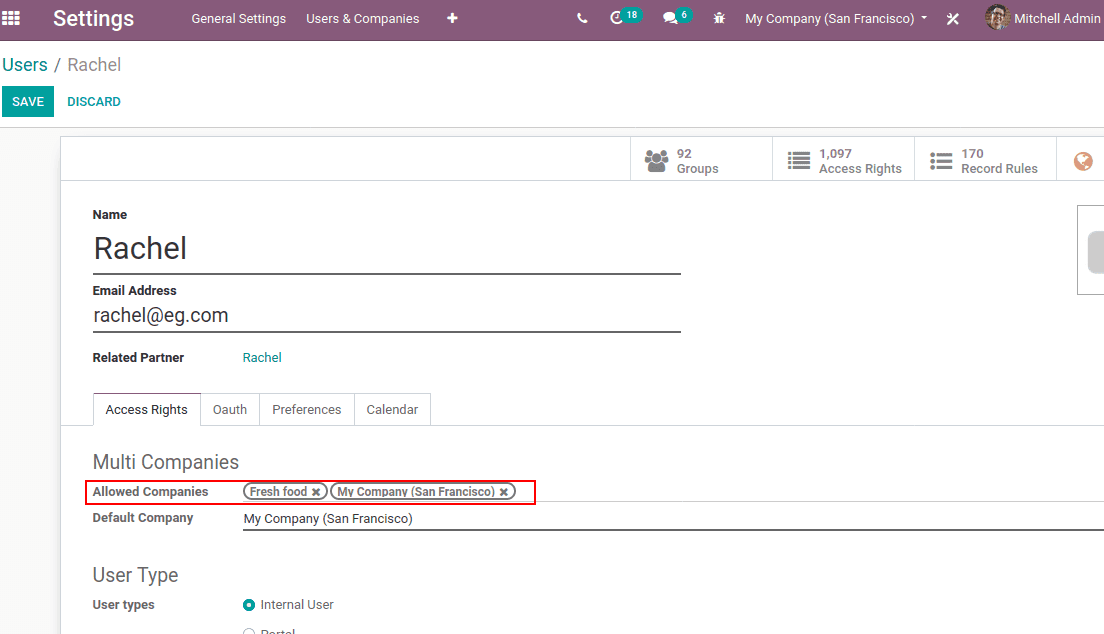The user profile interface displays detailed information from left to right. 

At the top left, the navigation options include "Settings," followed by "General Settings," and "Users and Companies." Adjacent to these, icons for add (+), phone, message, and an additional function are aligned. The label "My Company" is shown next to "San Francisco" in parentheses, accompanied by a tools icon.

The profile section features a picture of the profile holder alongside the name "Mitchell Admin." Below this main profile, a sub-section titled "Users" lists an individual named Rachel. Options to "Save" and "Discard" changes are available.

Rachel's profile highlights several attributes: 
- **Groups**: 92
- **Access Rights**: 1,097
- **Record Rules**: 170

Further, the detailed profile includes:
- **Name**: Rachel
- **Email Address**: rachel@eg.com
- **Related Partner**: Rachel

Below Rachel's information, four hyperlink options are available:
1. Access Rights
2. OAUTH
3. Preferences
4. Calendar

The displayed tab is "Access Rights," showcasing the following:
- **Multi-companies**: Allowed Companies
  - **Fresh Food**
  - **My Company San Francisco**
- **Default Company**: My Company San Francisco

At the bottom of the screen, the user type is indicated as "Internal User."